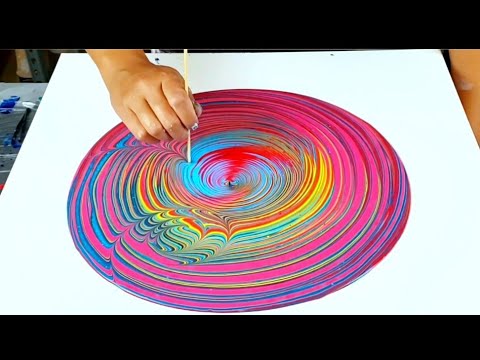In this meticulously framed photograph, a scene of artistic creation unfolds against a backdrop of perfect symmetry and vibrant hues. We observe an artist, whose hand extends gracefully from the upper left corner of the image, clutching what appears to be a slender wooden stick, reminiscent of a dowel or chopstick. Below, a pristine white canvas lies in focus, adorned with a mesmerizing array of colorful swirls that dominate the composition.

The artist seems to be employing a technique that involves the careful application and manipulation of paint. The colorful design features a series of concentric circles, crafted in a dynamic spectrum of colors, including deep blues, vivid reds, bright yellows, subtle pinks, and rich purples. The innermost circle showcases a blend of blue and red, while the outer rings favor hues of pink and blue. The swirling patterns suggest a method where paint is generously applied and then skillfully swirled using the wooden stick to create intricate, swirling designs that give the impression of motion and fluidity.

Despite the lack of visible equipment to spin the canvas, the detailed textures and harmonious blending of colors manifest an illusion of motion, enticing the viewer to ponder the innovative technique behind the artwork. The image is letterboxed, framing the rectangular canvas with black bands at the top and bottom, highlighting the central action and drawing the viewer’s eye to the artist's deft hand and the vibrant, swirling masterpiece in progress.